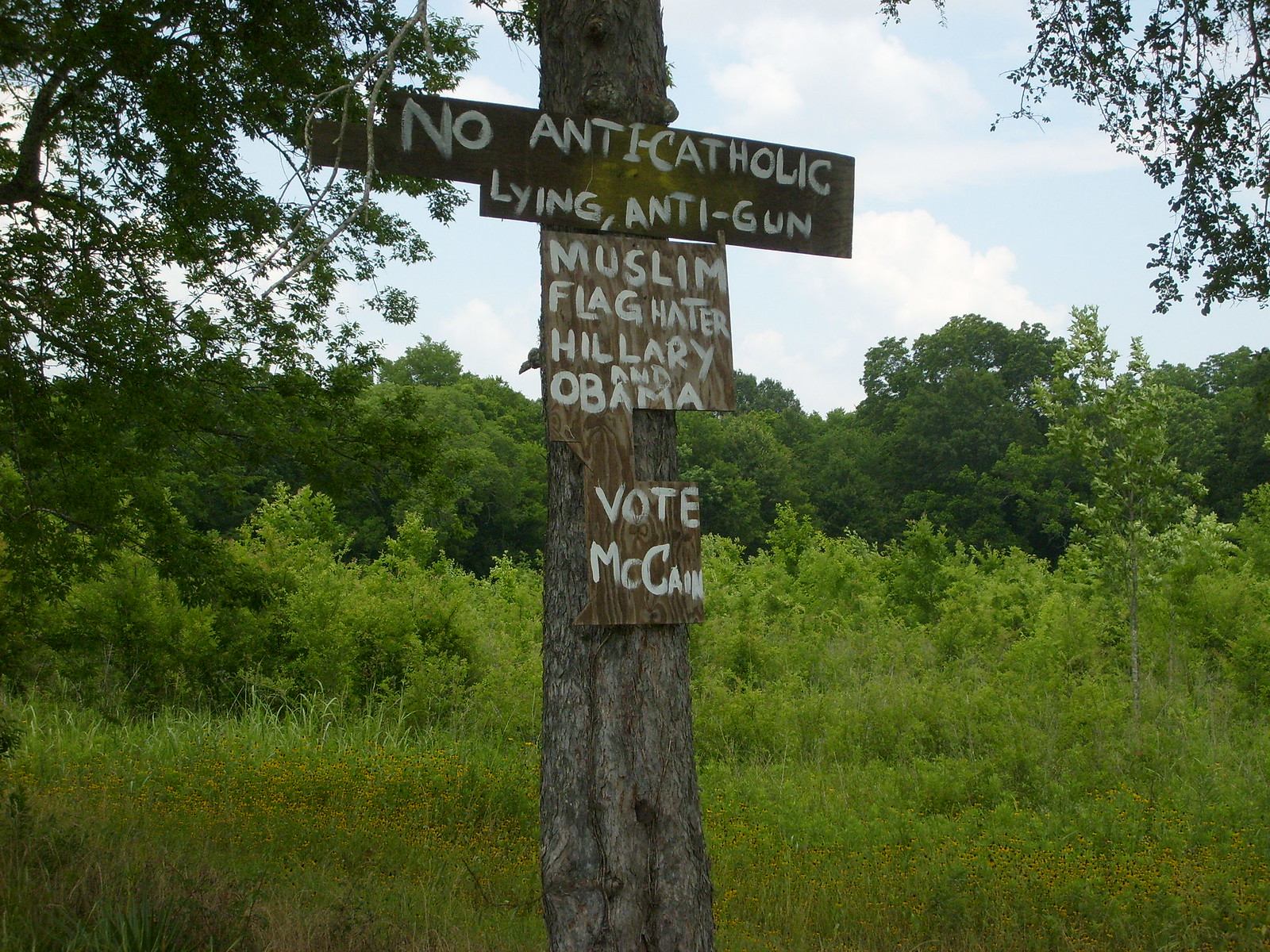In this image, a hand-painted political message is displayed on a tree located in a rural area. The tree is set amidst a lush green field, surrounded by other fully leafed trees and various shrubs, indicating the countryside setting. The message, written in white lettering and spanning three sections, conveys a strong political stance. The top section, wider than the tree itself, reads: "No anti-Catholic, lying, anti-gun, Muslim flag hitter, Hillary and Obama." The middle section, narrower and confined within the tree trunk, continues with an explanation of the accusations against Hillary and Obama. The smallest section at the bottom, also within the tree trunk, succinctly states: "Vote McCain." The choice of this remote, natural setting for a political sign is unusual, as its visibility is limited compared to more populated areas. Nonetheless, the sign's detailed, vehement message is clear in its advocacy.